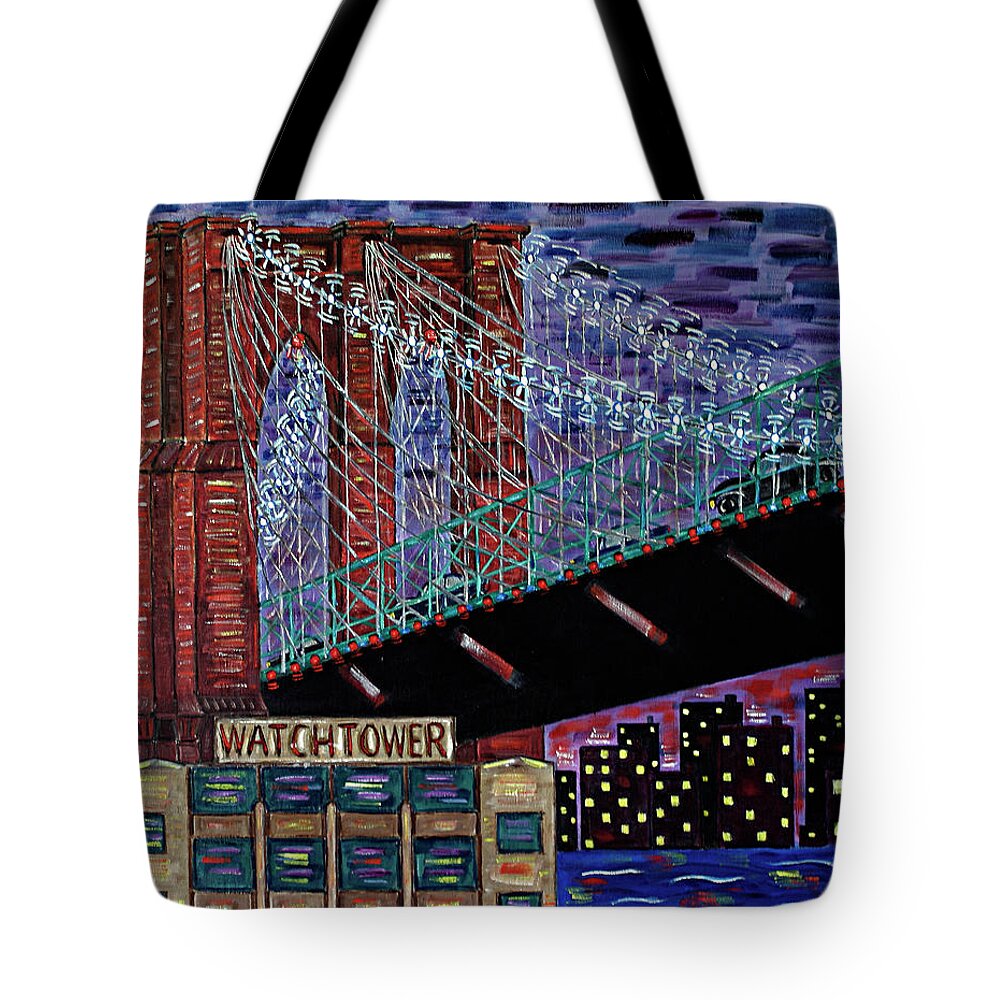This is an artist-designed purse featuring a hand-painted, abstract depiction of a red bridge with the word "Watchtower" inscribed below it. The bag showcases various elements that stand out: the top and right edge are blue, while the left side displays vivid red. The scene includes concrete supports of the bridge and a series of black buildings with illuminated windows beneath it, suggesting a city skyline. The water below the bridge contrasts with a mixture of white lines, yellow dots, red dots, and green dots, creating an abstract effect. A pink sky hovers over the cityscape. The bag has a large black strap at the top for carrying. The artistic composition integrates muted tones of dark blue, black, and purple, blending seamlessly to create a visually striking and unique accessory.